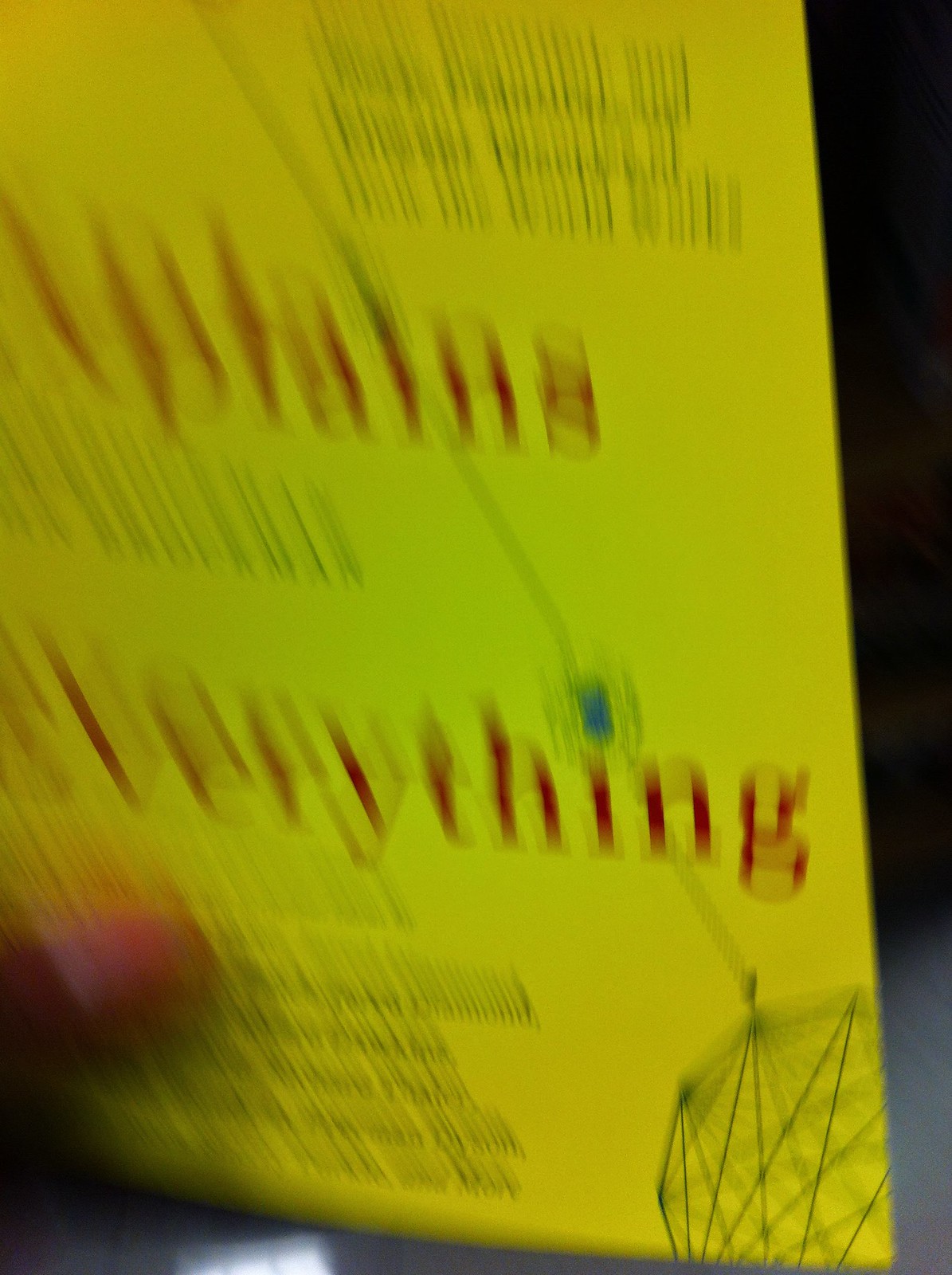The image depicts an angled, partial view of a yellow book cover that appears stretched and out of focus. The book's title is prominently displayed in red text, accompanied by smaller black text in various locations, including a section in the top right and another section interspersed between the red title. Towards the bottom of the cover, more black text can be seen, and in the bottom right corner, there is a circle design featuring intersecting lines. A person's thumb is visible on the bottom left of the image, resting on the book cover with their fingers positioned behind it. The edge of the book is visible at the top right, with a dark and indistinct background beyond it.